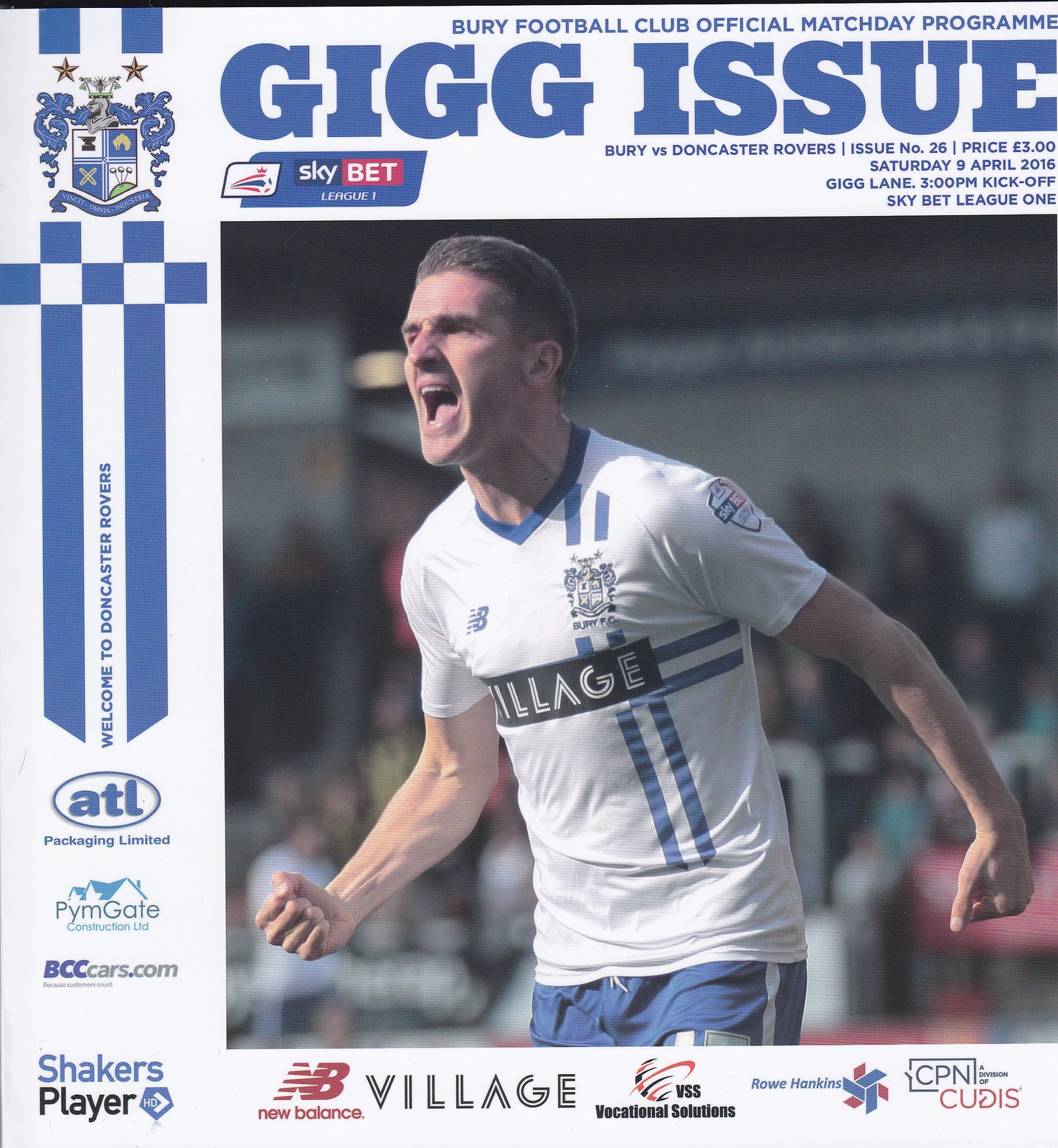This image is the cover of the official matchday program for a Sky Bet League One game between Bury Football Club and Doncaster Rovers. Positioned prominently at the top are the details: "Bury Football Club Official Matchday Program," "GIGG Issue," "Bury vs. Doncaster Rovers," "Issue No. 26," "Price £3," and the date and time – "Saturday, 9 April 2016, GIG Lane, 3pm kick-off." 

Centrally, a dynamic action shot captures a jubilant football player clad in a predominantly white jersey with blue accents and the word "Village" emblazoned across the front. The player, wearing blue shorts, is depicted mid-celebration, mouth open and fists clenched, channeling the energy and excitement of the game.

Surrounding the central image is a plethora of advertisements and logos from sponsors such as ATL Packaging Ltd., Pimgate, and BCC Cars. On the left side, adjacent to the player, there is a vertical banner featuring the club's heraldic shield, which consists of blue and white checkerboards and elaborate embroidery. Additional sponsors' logos are also positioned near the bottom of the cover, collectively framing the scene and adding to the visual structure of the program.